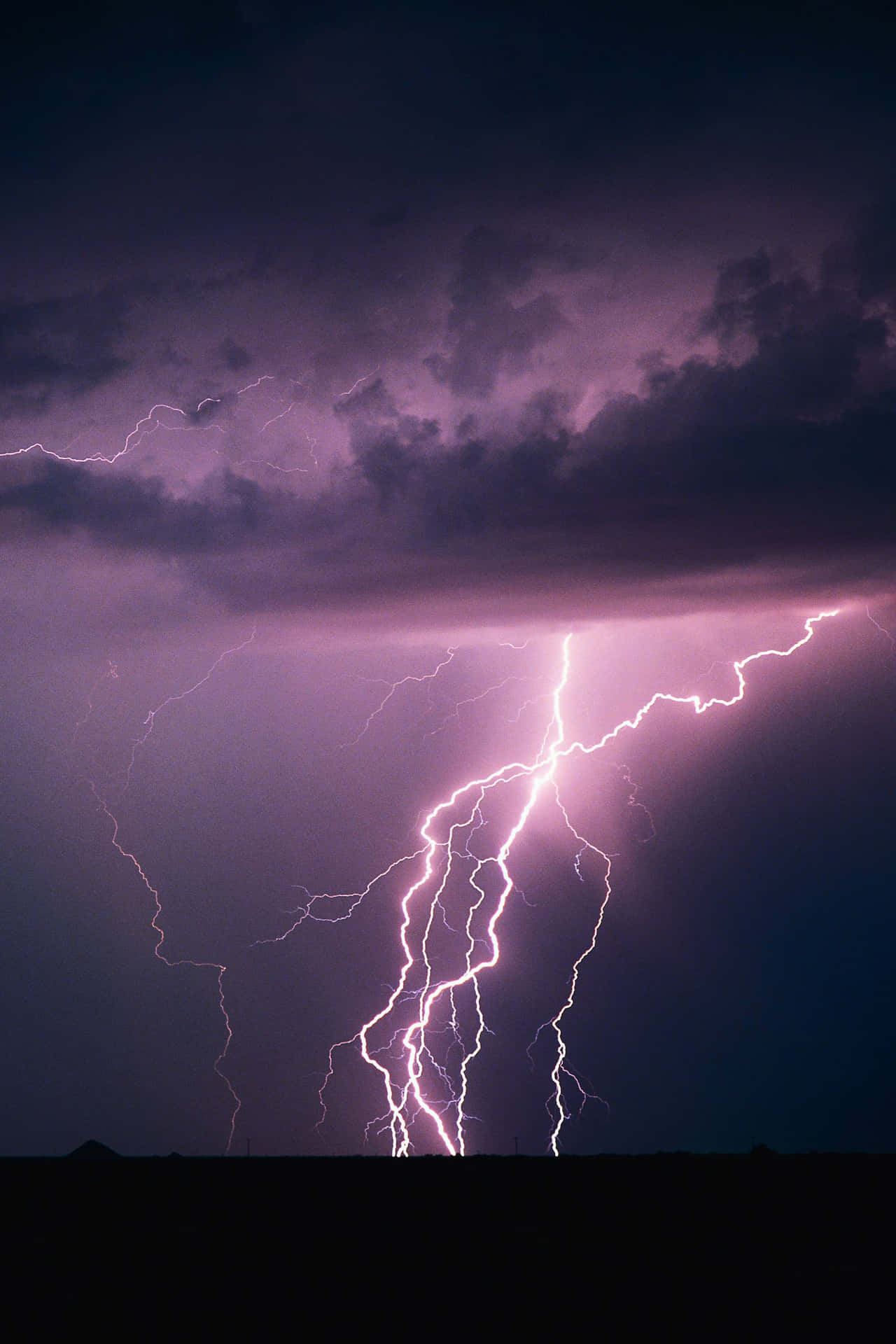This photograph captures an intense nighttime thunderstorm, vividly showcasing multiple bolts of lightning striking from the dark, heavy clouds down to the ground. The sky features an array of colors, transitioning from deep purples and dark blues to lighter hues of purple, with patches of hot pink and bright white where the lightning is most intense. The image's base is a solid black, possibly indicating silhouettes of objects like rooftops, though they are indistinct. The dark, nearly black clouds starkly contrast with the lightning, which zigzags through the sky, creating a mesmerizing and dramatic scene. There are several exceptionally bright lightning bolts illuminating the entire sky, surrounded by fainter, more diffused lightning, all contributing to the electrifying atmosphere of this powerful storm.